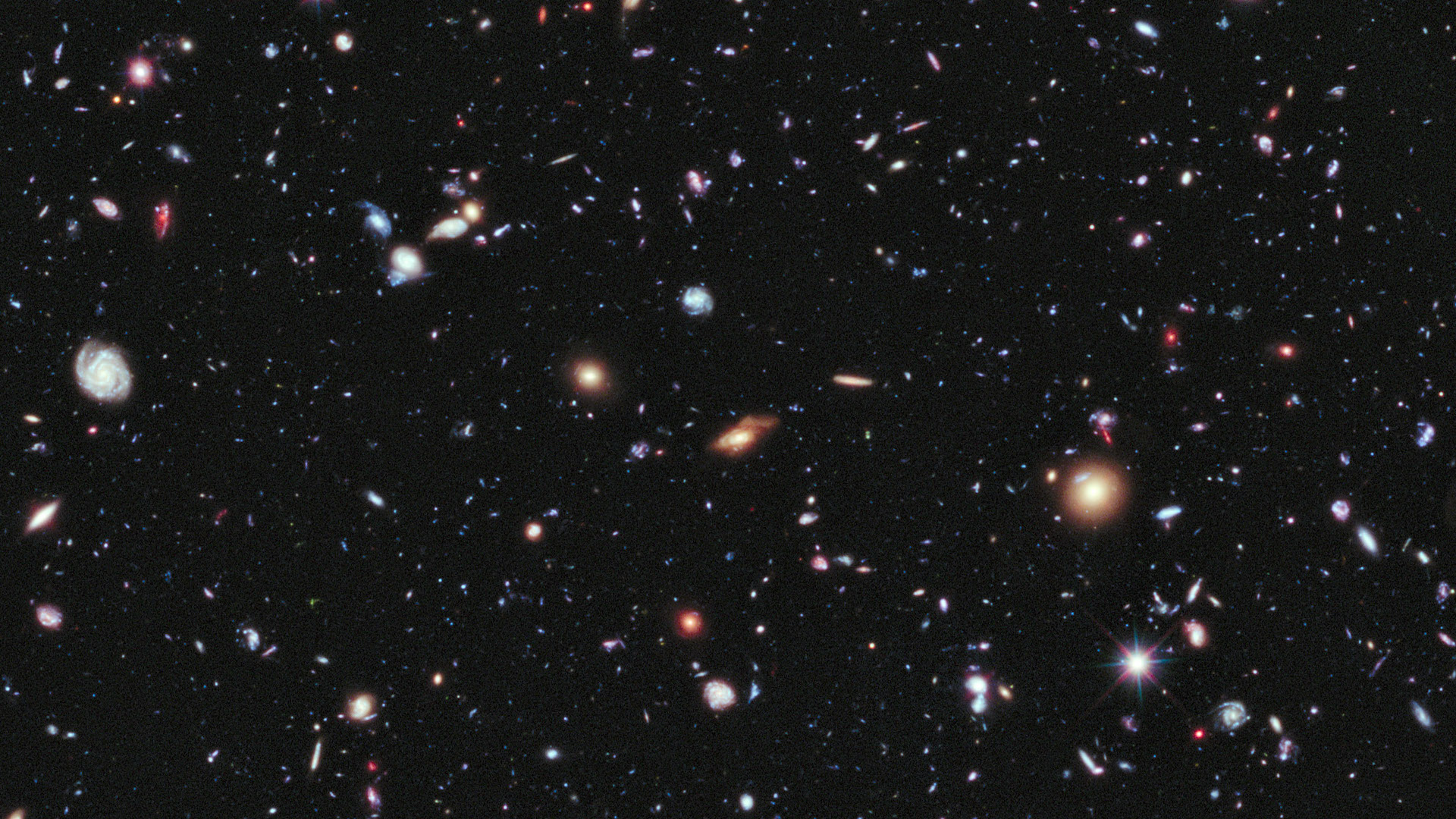This full-color, horizontally rectangular photograph taken outdoors in space captures the vastness of the universe, showcasing the famous Hubble Deep Field image. The background is the profound blackness of space, speckled with countless galaxies, each varying in size and color, highlighting their distances from us. The image reveals intricate details of spiral galaxies in shades of red, yellow, white, orange, and blue. Among these galaxies, smaller pinpricks of light represent entire galaxies with billions of stars. The photograph might also include a few stars from within our own galaxy, mixed among the more distant celestial objects. The captivating colors and the sheer number of visible galaxies underscore the immense scale and beauty of the cosmos.